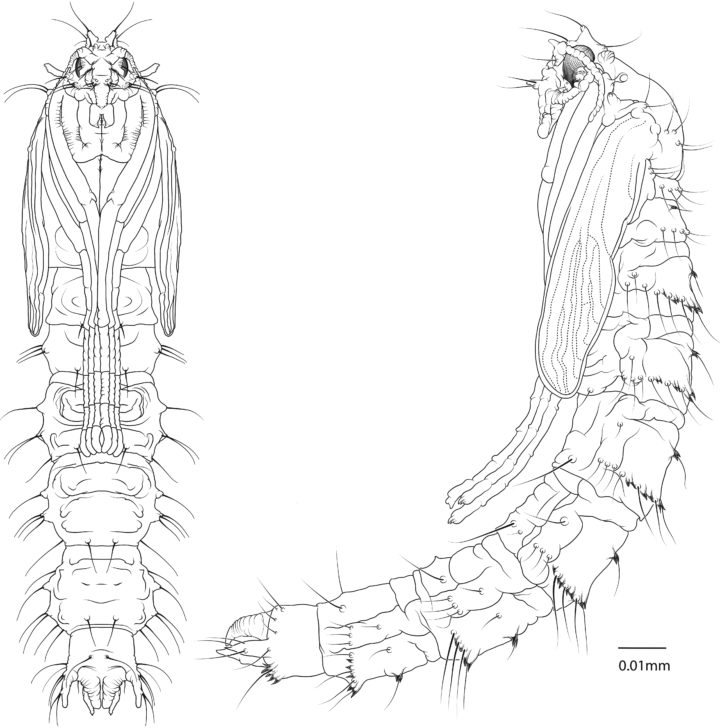This is a detailed black and white, hand-drawn illustration, likely done in pencil, depicting a caterpillar or an insect larva. The drawing appears to be from a textbook or a scientific reference book. The main image shows a vertically-oriented view of the caterpillar from its underside, revealing numerous small appendages, perhaps antennae or tentacles, with an estimated 20 on each side. Adjacent to this is a side view of the same creature, featuring a prominent black eye and facial features that might suggest a nose and chin, giving it an almost anthropomorphic appearance. This detailed depiction includes an annotated scale at the bottom right, indicating a microscopic examination with a measure of 0.01 millimeters. The caterpillar also has vestigial wings on the sides, though it is uncertain if they enable flight, and the overall shape of the body is long and oblong, with curved segments.